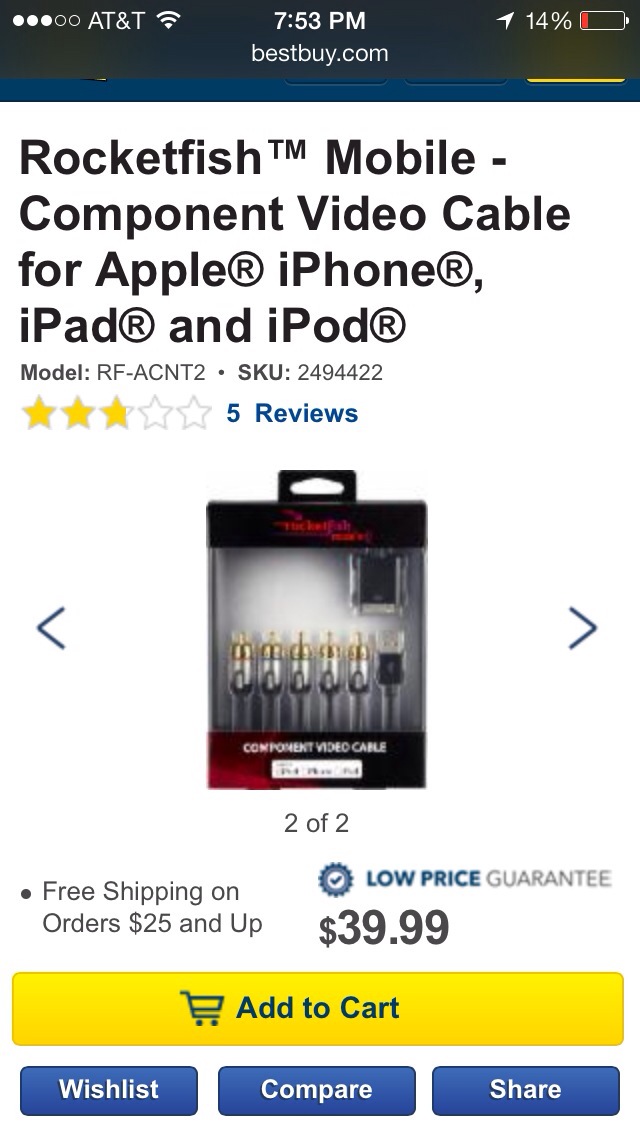The screenshot captured on a phone at 7:53 p.m. under AT&T service shows the BestBuy.com webpage with a 14% battery indicator. The screen features a Rocketfish™ mobile component video cable compatible with Apple iPhone, iPad, and iPod devices. This product has a mixed rating of three stars based on five reviews. Priced at $39.99, the listing includes a low price guarantee and an offer for free shipping on purchases over $25. The displayed image prominently features the five cables, mostly gold in color, within their packaging. Navigation arrows beside the image allow for viewing additional pictures. Below the product description, there are interactive buttons: a yellow "Add to Cart" button, and blue "Wishlist," "Compare," and "Share" buttons, providing various options for potential buyers.